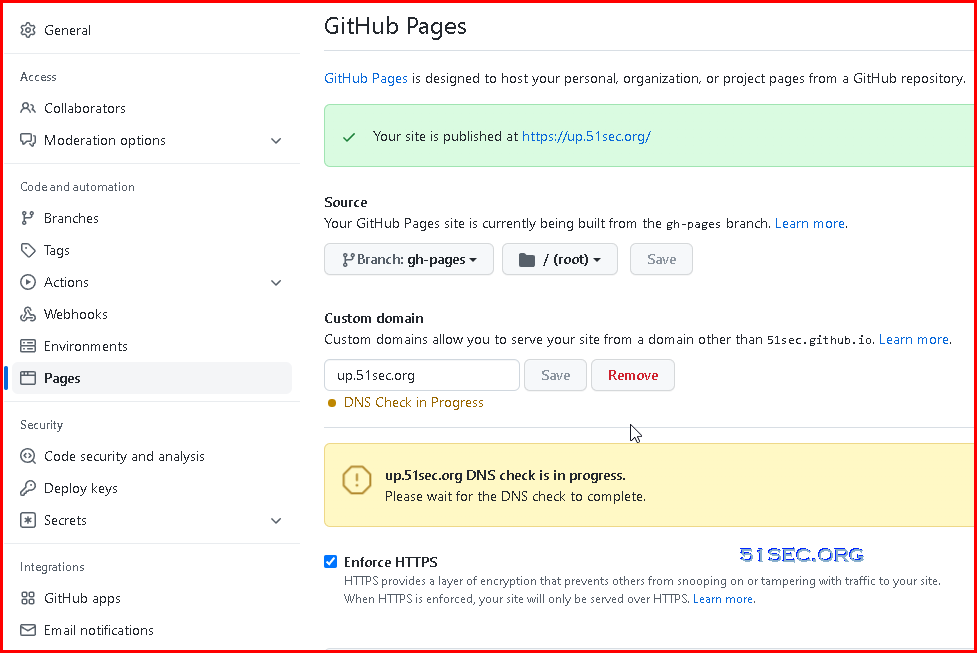Screenshot of GitHub Settings

This image captures a detailed view of the GitHub Pages settings within a GitHub repository. At the top, it prominently displays a section header that reads, "GitHub Pages," along with a brief description: "GitHub Pages is designed to host your personal, organization, or project pages from a GitHub repository."

On the left side of the screenshot, there is a navigational sidebar featuring various categories and options that users can access to modify their GitHub Pages settings. The categories and their respective options are listed as follows:

1. **General**
2. **Access**
3. **Collaborators and Moderation Options**
4. **Code and Automation**:
   - Branches
   - Tags
   - Actions
   - Webhooks
   - Environments
   - Pages
5. **Security**:
   - Code Security Analysis
   - Deploy Keys
   - Secrets
6. **Integrations**:
   - GitHub Apps
   - Email Notifications

In the middle section of the screenshot, there is a highlighted message indicating that the site is published and available at a specific URL. This section includes:

- **Published Site Link:** A clickable link indicating where the site is live.
- **Source:** Information about the source branch for GitHub Pages.
- **Root File:** Details concerning the root directory for the pages.
- **Custom Domain:** A custom domain is specified as "up.51sec.org," with an alert message noting that a DNS check is currently in progress. This alert is displayed with yellow text on a background meant to catch the user's attention.

Overall, this screenshot provides a comprehensive overview of the various settings and configurations available for GitHub Pages, along with specific details about the current state and custom domain status of the user's published site.